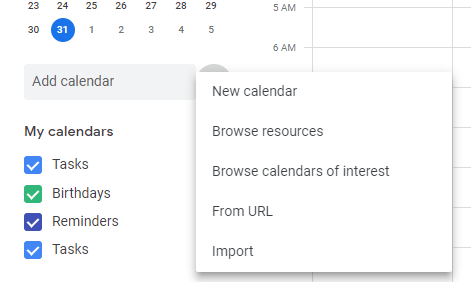This image features a digital calendar interface set against a white background. At the top left corner, the dates 23, 24, 25, 26, 27, 28, and 29 are displayed in a single row. Below this row, the date 30 is shown, followed by the date 31, which is encircled in blue. Proceeding downward, the dates 1, 2, 3, 4, and 5 are aligned consecutively. Beneath these dates, against a gray backdrop, the text "Add Calendar" is prominently displayed.

On the left side of the page, a section labeled "My Calendars" is visible. Here, a blue box with a white checkmark is labeled "Tasks." Adjacent to this, a green box with a white checkmark is next to the word "Birthdays," followed by a purple box with a white checkmark next to the word "Reminders." Notably, another blue box with a white checkmark appears next to the word "Tasks" again.

On the right side of the page, time slots are listed vertically, starting with "5 a.m." and "6 a.m.," each accompanied by a horizontal line. These lines segment the hours, although no additional text or events are displayed within these times.

Further down the page, a white rectangular box contains a series of text lines in the following order from top to bottom: "New Calendar," "Browse Resources," "Browse Calendars of Interest," "From URL," and "Import." Beyond this text-containing rectangle, the page is notably devoid of any photographs, drawings, or additional markings.